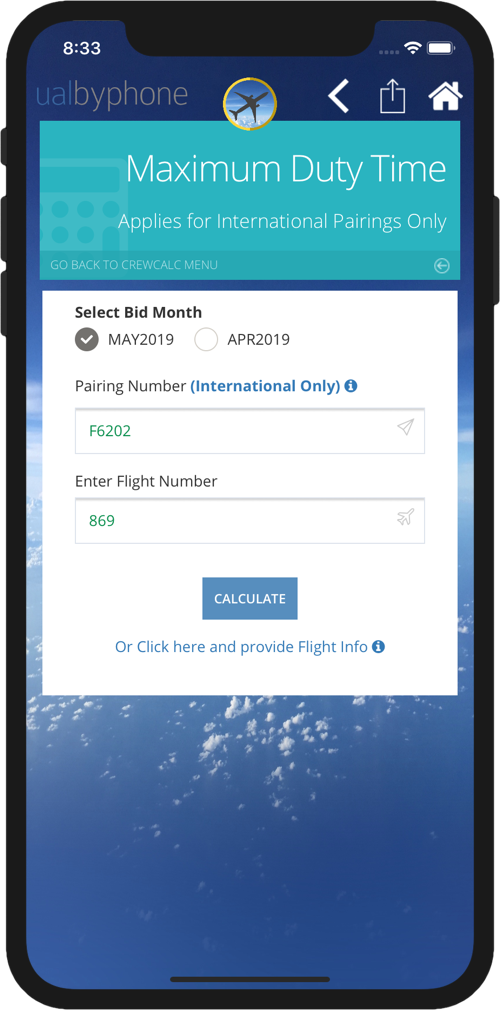The image showcases a mobile application interface designed to calculate maximum duty time for international flight personnel. At the top left of the screen, the current time is displayed as 8:33, although it does not specify whether it is a.m. or p.m. This image appears to be a sample taken from a mobile phone, likely an iPhone, though it could be from any generic smartphone.

The app is identified with the name "UL by phone," featuring a logo of an airplane, indicating its association with United Airlines. Toward the top right corner of the interface, there are navigation icons, including a home button for returning to the main menu and a share icon for distributing information to other apps or services. These icons are positioned just below the top right corner.

The main content of the screen is centered around the calculation of maximum duty time. It prominently displays the heading "Maximum Duty Time" and offers an option to select a bid month, with "May 2019" currently selected.